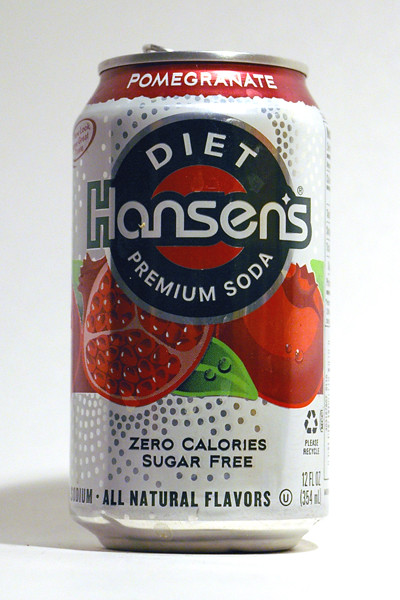This is an image of a soda can set against a gradient background transitioning from gray to white, with a darker gray shadow on the left and a bluish tint at the bottom. The can itself has a silver top and is primarily white with a prominent red section at the top featuring the word "pomegranate" in white letters. In the center of the can, there is a large circular logo with a silver border. Inside the circle, the top portion is blue with the word "diet" in white letters, and the middle is red with "Hansen's" in white letters outlined in blue. The "H" has a greenish outline. Below this, also within the blue circle, it says "premium soda." The background of the can shows illustrations of pomegranates, including one partially cut open, accompanied by green leaves. Scattered across the white part of the can are silver and blue dots. Near the bottom, the text "zero calorie," "sugar free," and "all natural flavors" is written in black. Additionally, there is a circular symbol with a "U" inside it and a recycling logo. On the lower right side, it says "12 FL OZ" followed by smaller, unreadable text.